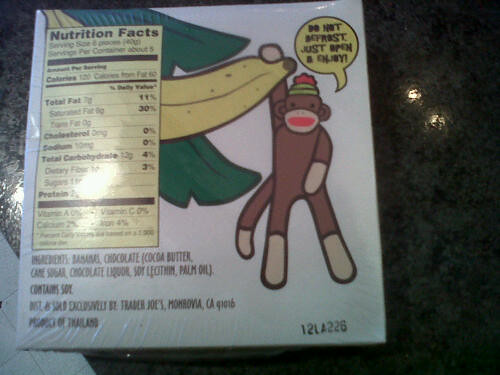This image showcases the back of a food product package featuring a vividly illustrated scene with a playful sock monkey hanging from a large banana. The sock monkey, which is brown with beige feet and tail tip, clings to the banana with one arm, appearing lively and dynamic against the backdrop. There are also two vibrant green banana leaves adding to the tropical theme. Overlaying this playful illustration is a Nutrition Facts label, which is prominently placed in a yellow box with black text. Although some details are obscured due to glare and blurriness, you can discern key nutritional information: serving size, calories (120), total fat (7 grams), cholesterol (0 grams), sodium (10 milligrams), total carbohydrates (13 grams), and protein. The ingredient list includes bananas, chocolate, cocoa butter, cane sugar, chocolate liqueur, soy lecithin, and palm oil, and it notes that the product contains soy and is manufactured exclusively for Trader Joe's. There is also a barely readable speaking or thought bubble near the sock monkey, adding a whimsical touch to the packaging. The product is displayed against a dark green marble-like surface, with the code 12LA226 printed on the bottom right corner of the package.